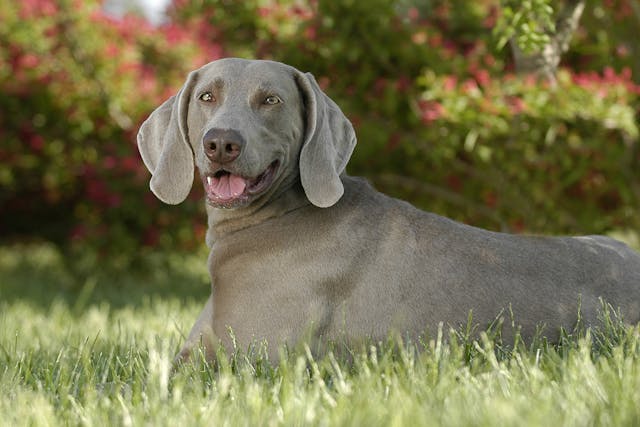A medium to large-sized, muscular gray dog, resembling a Labrador or retriever, is sitting gracefully on a patch of tall, vibrant green grass. The dog's short coat glistens under the clear, sunny sky. His big, wet, dark brown nose and light green eyes add a striking contrast to his appearance. His pink tongue hangs out of his mouth, indicating perhaps a moment of play or rest. Long, floppy ears frame his attentive face as he sits in front of a lush backdrop of tall shrubs adorned with fuchsia-colored flowers. A sliver of blue sky peeks through in the background, completing this picturesque scene.